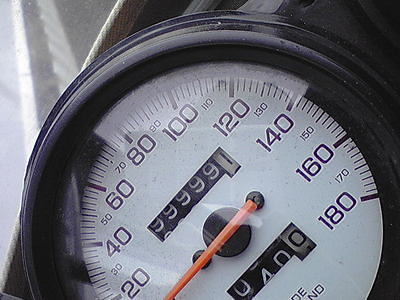The image features a detailed view of a vehicle's speedometer and odometer. The speedometer displays large, clear numbers indicating kilometers per hour, with increments marked at 20, 40, 60, 80, 100, and so on, up to 180 km/h. The smallest visible number is 20 km/h, while the largest is 180 km/h, with additional smaller numerals marking every 10 km/h interval, such as 30, 50, etc. Notably, the dial appears slightly tilted to one side.

The odometer, located at the top of the dial, indicates a high mileage reading of 99,999.1 kilometers. Below it, a trip meter shows a reading of 40 kilometers. A red arrow pointer on the speedometer indicates the current speed of the vehicle. The entire display is encased in a circular plastic rim, providing a clear and organized view of all the instrumentation.